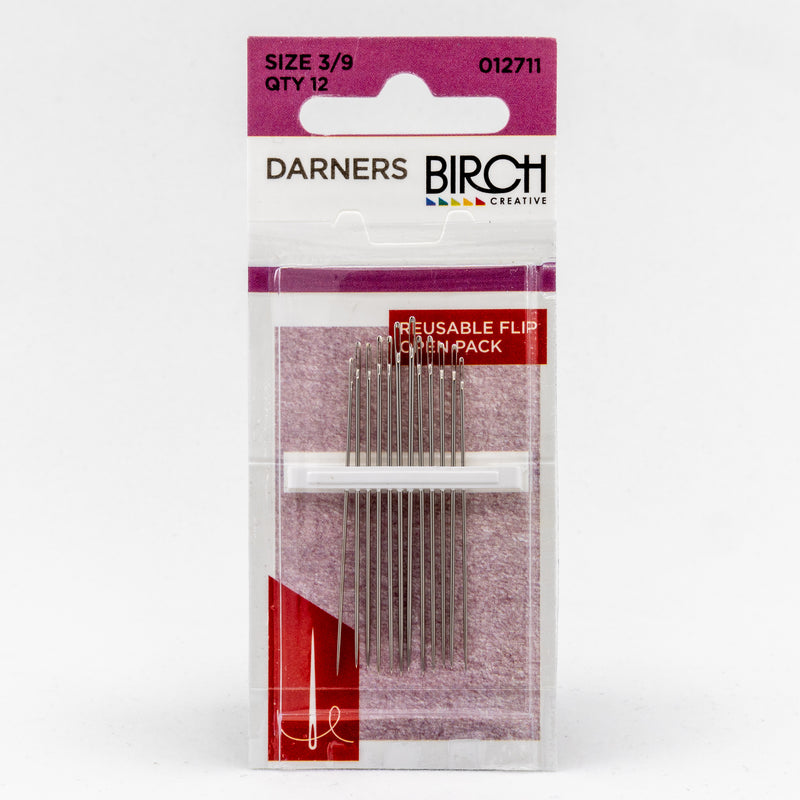This image displays a package of sewing needles set against a plain white background, typical of a product listing on an e-commerce site. The package is a rectangular, clear plastic blister pack with a dual-colored design, featuring a purple stripe at the top and a white bottom section. At the top of the package, a purple tab highlights essential product details: "Size 3/9" in black font, "QTY 12" below that, and "012711" in the top right corner. The tab also includes a hole for hanging on a store display rack.

The main body of the packaging prominently displays the brand "Darners Birch Creative" alongside a small, multicolored logo on the left. The bottom right corner features an image of a sewing needle with red and white accents, and a label reading "Reusable Flip Open Pack." The transparent portion of the blister pack clearly shows all 12 sewing needles inside, emphasizing their orderly and present arrangement. This attention to detail and presentation indicates the product’s readiness for retail display and online sale.